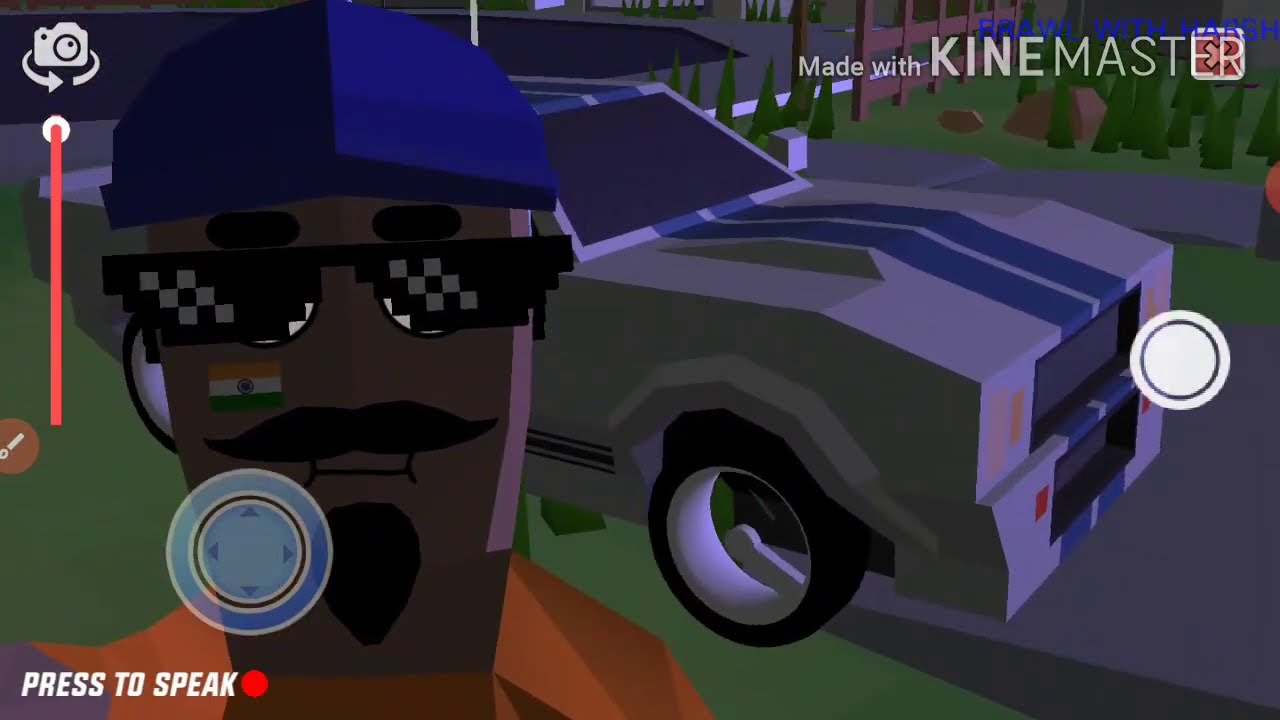The image appears to be a computer-generated rendering, possibly from a video game or design program. Dominating the left side of the image is a man resembling a Lego figure, characterized by pixelated black sunglasses, a blue hat, and a prominent goatee and mustache. Notably, he has a green, yellow, and white flag with a blue circle underneath his right eye. He is dressed in an orange shirt and is facing the viewer. Behind him is a sleek, white or gray car adorned with two blue stripes extending from the front to the back. The background features a road, trees, a fence, and rocks, all rendered in a CGI style. In the bottom left corner, the text "Press to Speak" is displayed alongside a red circle, while in the top left, there is a camera icon with a rotation symbol, suggesting a 3D viewing capability. The top right corner includes text that reads "Brawl with Harsh, made with Kindmaster," indicating the software or platform used for creating the image. The color palette includes various shades of black, white, gray, blue, red, orange, tan, and green, yet the image lacks clear context regarding its overall narrative or purpose.